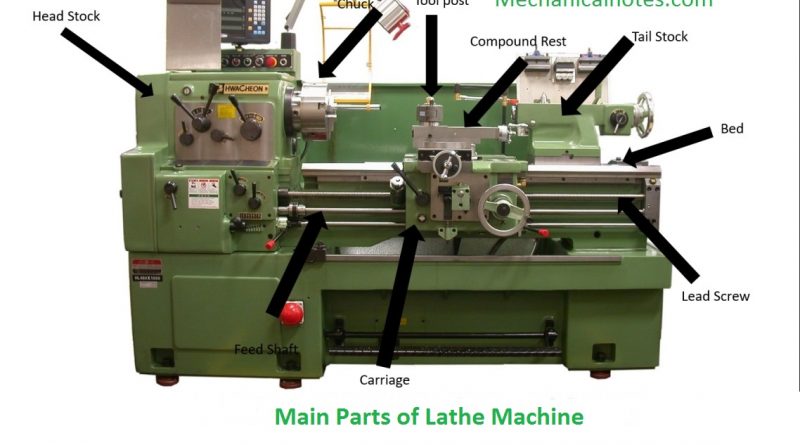This highly detailed illustration of a lathe machine appears to be taken from a technical encyclopedia or dictionary. The large, green machine is depicted with numerous intricacies, featuring various metallic silver components such as levers, gears, and a steering wheel on the right side which is used to control its functions. Prominent black arrows are meticulously directing attention to the key sections of the lathe, including the headstock in the upper left, chuck, tool post, and compound rest near the top, and the tailstock in the upper right. The middle and lower portions of the machine identify the bed, lead screw, and carriage, with the latter positioned towards the center by arrows labeled "feed shaft." Additionally, a notable red button is situated above the feed shaft. This image is topped with the title "Main Parts of a Lathe Machine" in bluish-green text at the bottom, firmly distinguishing each element of the machine to provide comprehensive detailing for educational purposes.